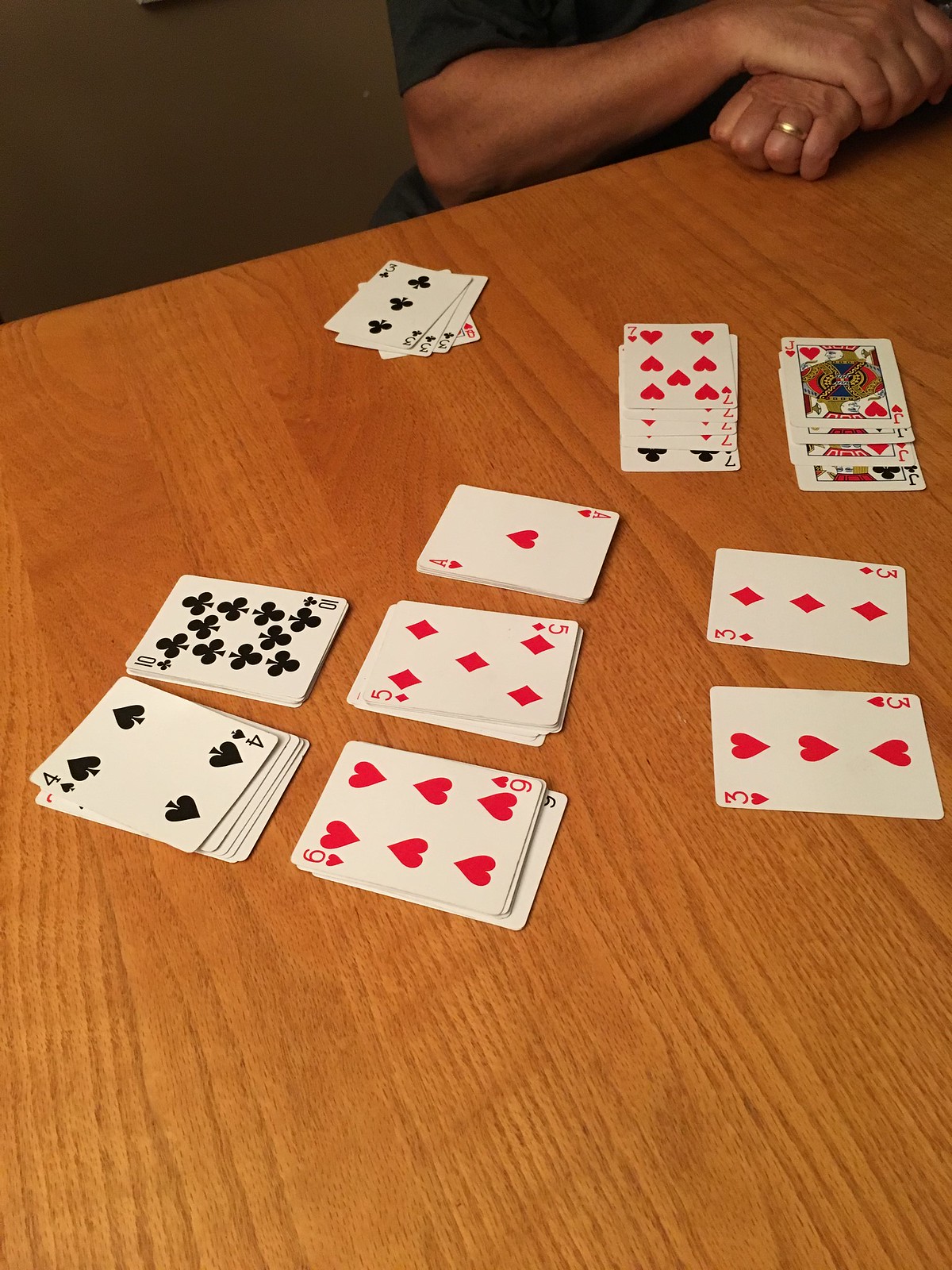This image showcases a moment during a card game, set on a rich, brown wooden table with visible grain running diagonally from the bottom right to the upper left corner. In the upper right section of the image, a person is seated with their hands folded. The right hand rests over the left, which is laid flat on the table with fingers curled under. A gold wedding band is noticeable on their left ring finger. The individual, likely male, wears a dark t-shirt with visible cuffs revealing only the forearms and hands. 

Their right hand covers the back of the left, with fingers curled down, creating a bent position at the wrist. Beneath the table, a hint of dark fabric, possibly from the person's pants, is visible. 

On the table in front of this person are several stacks of playing cards. Prominently, four jacks are lined up, one on top of the other, just in front of their hands. To the left of these jacks is a stack of sevens. Near the center and slightly towards the upper left, a small discard pile exists, nearly at the table's edge, consisting of three threes and a queen underneath. 

The arrangement of cards also extends from the left with sequential placements: a three of diamonds, a three of hearts, then an ace of hearts, a five of diamonds, a six of hearts, a ten of spades, a ten of clubs, and a four of spades. Beneath many of these cards are more layers, indicating an ongoing strategic card game played on the wooden surface.